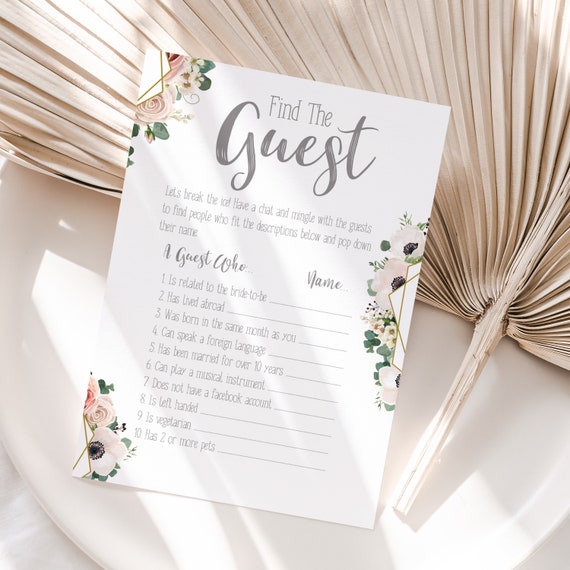This is a color photograph of a rectangular white printed wedding card, placed against a white ceramic plate. Behind the plate is a pleated, peach-colored hand fan shaped like a fan palm frond, made out of a light fabric material. The card is decorated with pink flowers and green leaves in the upper left corner, lower left corner, and the middle of the right edge. The card features gray text, with the bold header "Find the Guest" at the top. Below this, there are smaller text paragraphs that include instructions for the game: "Let's break the ice and have a chat and mingle with the guests to find people who fit the descriptions below and pop down their name." A list follows with ten numbered prompts such as "is related to the bride-to-be," "does not have a Facebook account," and "has two or more pets," designed to encourage interaction and conversation among guests at the wedding.